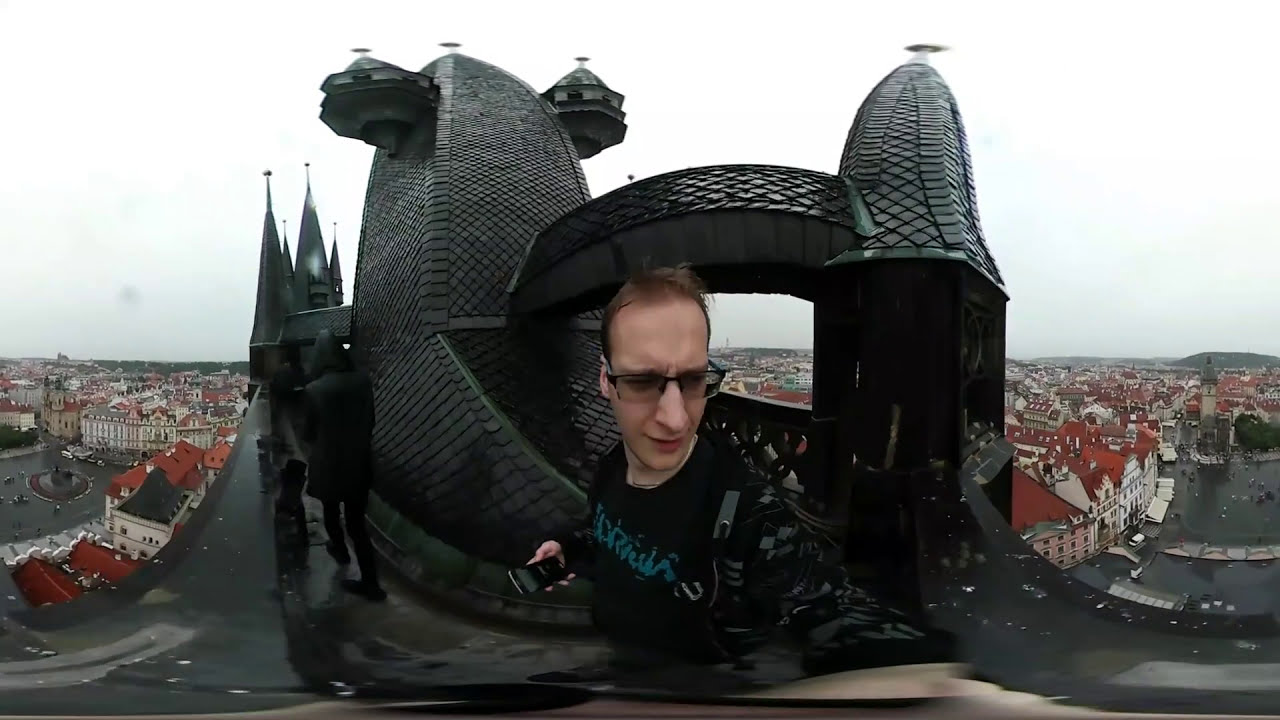The image is a manipulated panoramic shot featuring a young Caucasian man with short brown hair and black reading glasses, holding a phone in his right hand. His torso faces slightly to the left while his head looks directly at the viewer, displaying a confused expression. The photo has been distorted by a filter or lens effect that warps the structures and people within it, bending and bowing them in various areas.

Behind the man, there's an intricate black building resembling overlapping dragon or snake scales, contributing to the image's surreal appearance. This structure features two rounded-top towers connected by a dark brown and black walkway. To the left of this building, a man in a black hood and coat walks up a dark pathway next to several black spires, with other people also visible on this path.

Overlaying this scene is a small village with uniform off-white buildings topped with maroon roofs. In the background, beyond the village, a partly cloudy sky can be seen. The townscape includes greenery on the left and hills on the right, completing the picturesque backdrop. The warped effect melds these various elements together, creating a striking contrast between the distorted foreground and the serene, unaltered village behind.